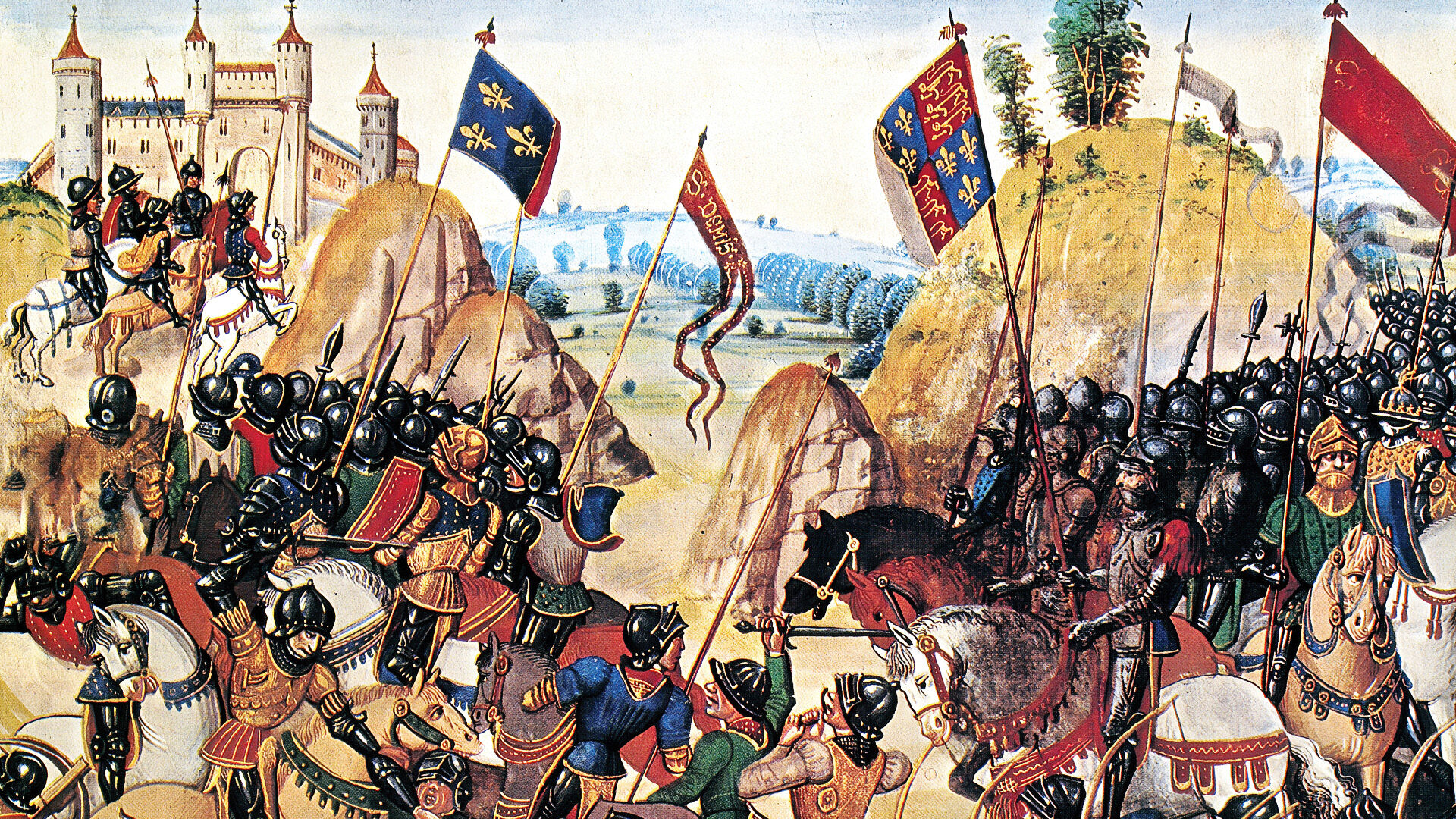The image is an ancient, vividly detailed painting of a medieval or possibly early modern battle scene featuring heavily armored cavalry troops, likely from a Spanish army due to their distinctive black helmets. Soldiers clad in a varied array of blue, green, red, and black armor are prominently displayed, riding identical horses across a field characterized by bumpy, elevated mounds with trees atop them. The scene bristles with the energy of clashing armies, some of whom wield swords, spears, and javelins while hoisting banners and emblems evocative of knighthood. In the backdrop, a towering castle, reminiscent of those from hundreds of years ago, looms over the chaotic yet vibrant tableau. The rugged terrain with hills and scattered trees, combined with a lightly white-colored sky, frames the multitude of troops—possibly numbering in the hundreds—moving in an expansive formation across the landscape.